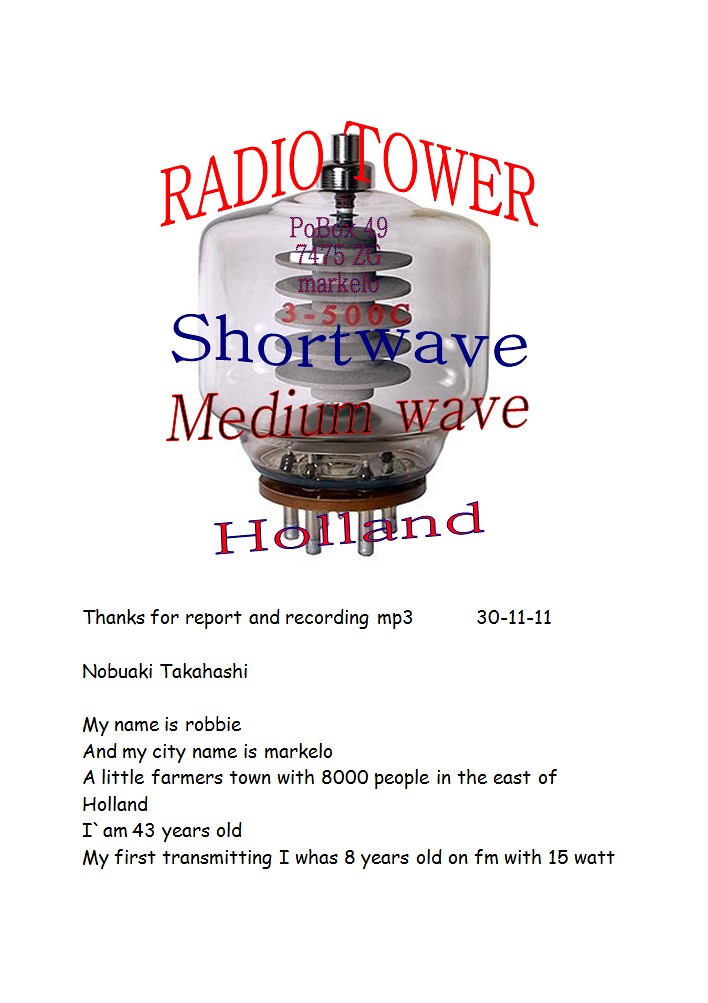The image features a digitally-rendered poster with a white background. Dominating the center is a peculiar light bulb-like structure, which closely resembles a vacuum tube. This structure is composed of five off-white, cylindrical discs stacked atop one another, encased within a glass bulb. At the base, brown and black metal prongs extend downwards.

Overlaying the image, the topmost section features the text "Radio Tower" in red. Below it, there are various lines of text in multiple colors: "PO Box 49-7475-2G Markello" in purple, "3-500C" in red, "shortwave" in blue, "mediumwave" in red, and "Holland" in red. 

Beneath the graphic, in plain black text, it reads: "Thanks for your report and recording, MP3-30-11-11. Nobuaki Takahashi. My name is Robbie, and my city name is Markello, a little farmer's town with 8,000 people in the east of Holland. I am 43 years old. My first transmitting, I was 8 years old on FM with 15 watts."